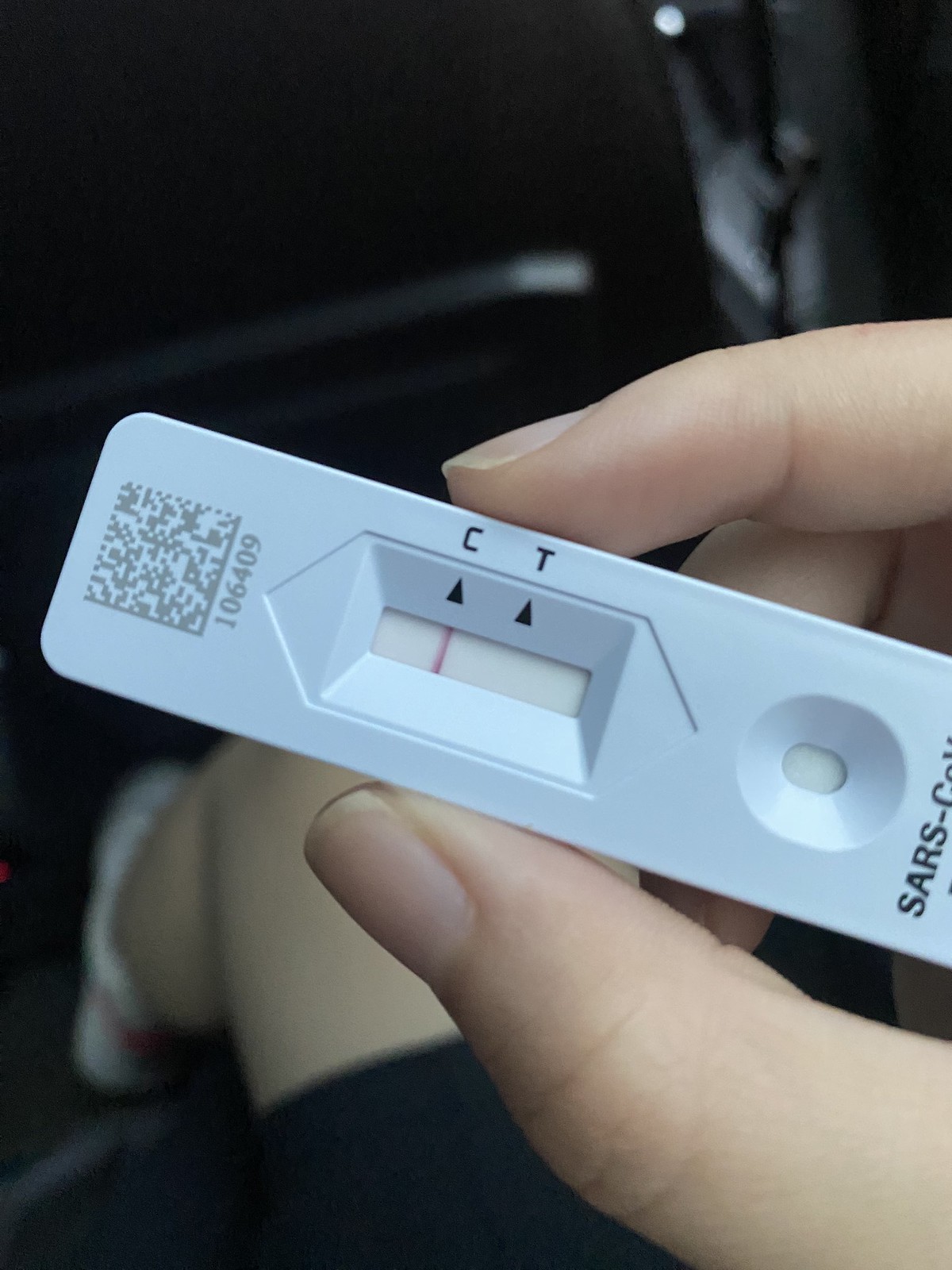A close-up image captures two fingers holding a blue COVID-19 test kit. The kit prominently displays the words "SARS COVID" in black lettering at the bottom. A QR code accompanied by a number is visible at the top of the kit. There is a single red indicator line running across the section marked with a "C" on the test kit. This detail suggests that the test has been completed and is indicative of the test result. Additionally, the lower half of the image reveals the legs of the individual holding the test kit, clad in black shorts, while seated in the back seat of a car.